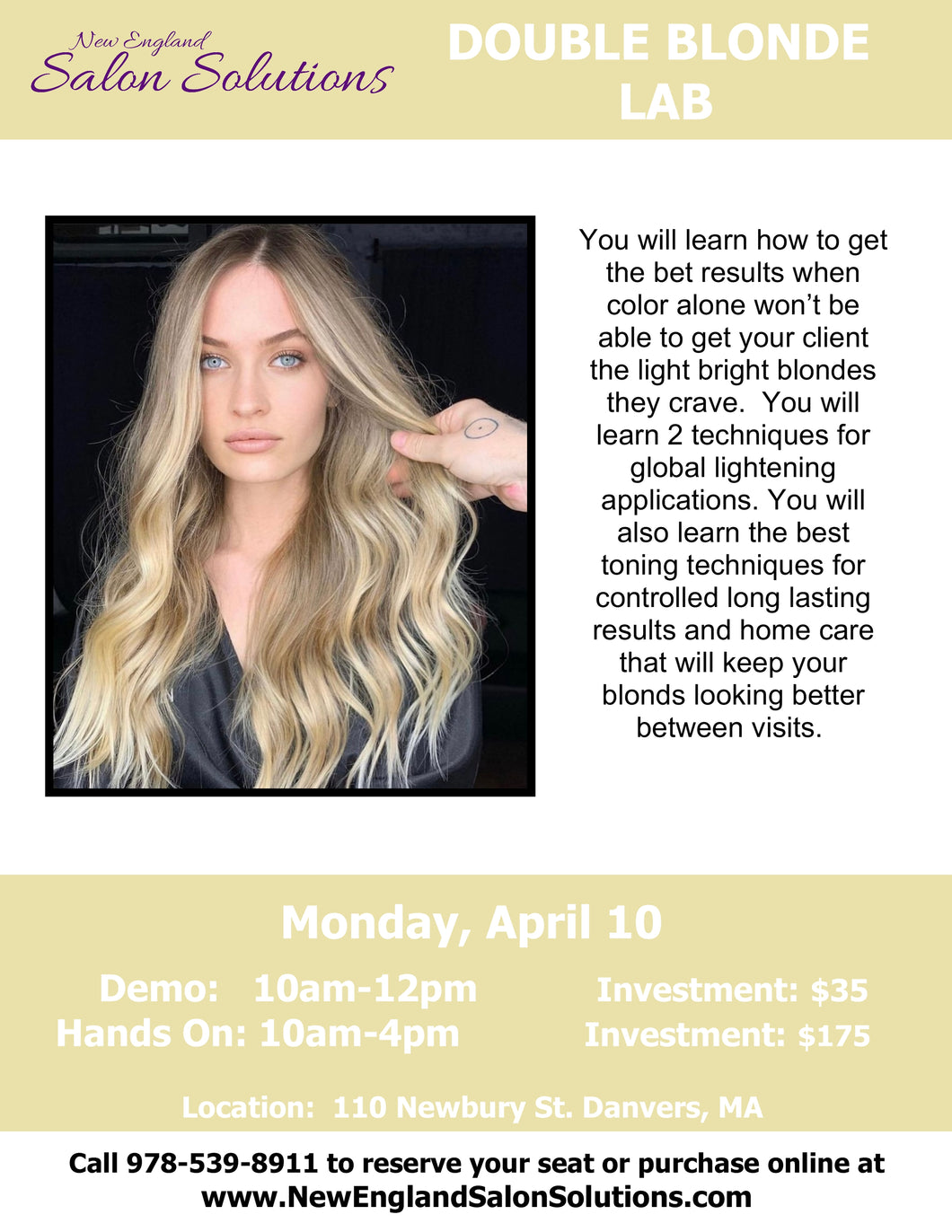This rectangular advertisement poster on a plain white background features details about an educational event hosted by New England Salon Solutions. The top section of the poster is highlighted with a gold-toned border that spans the entire width. In the upper left corner, "New England Salon Solutions" is displayed in elegant purple cursive, while "Double Blonde Lab" appears in bold white print to the right.

Below this header, on the left side of the poster, there's a photograph of a Caucasian woman with long, slightly wavy blonde hair parted in the center. A hand of similar complexion holds a section of her hair on the right, revealing the undertones. The woman, with blue eyes, is gazing directly at the camera.

To the right of the photograph, the text outlines the event's educational offerings in black print against a white background: "You Will Learn How to Get the Best Results When Color Alone Won't Be Able to Get Your Client the Light, Bright Blondes They Crave. You Will Learn Two Techniques for Global Lighting Applications. You Will Also Learn the Best Toning Techniques for Controlled Long-Lasting Results and Home Care that Will Keep Your Blonde Looking Better Between Visits."

Below this description, another gold rectangular section contains logistical information in white print. Centered at the top, it states "Monday, April 10th," followed by the schedule: "Demo 10 a.m. to 12 p.m." on the left with an "Investment $35" to the right, and "Hands-On 10 a.m. to 4 p.m." on the left with an "Investment $175" to the right. The location is listed as "110 Newberry Street, Danvers, Massachusetts."

At the bottom of the poster, contact information is provided in bold black print on a white background: "Call 978-539-8911 to reserve your seat or purchase online at www.NewEnglandSalonSolutions.com."